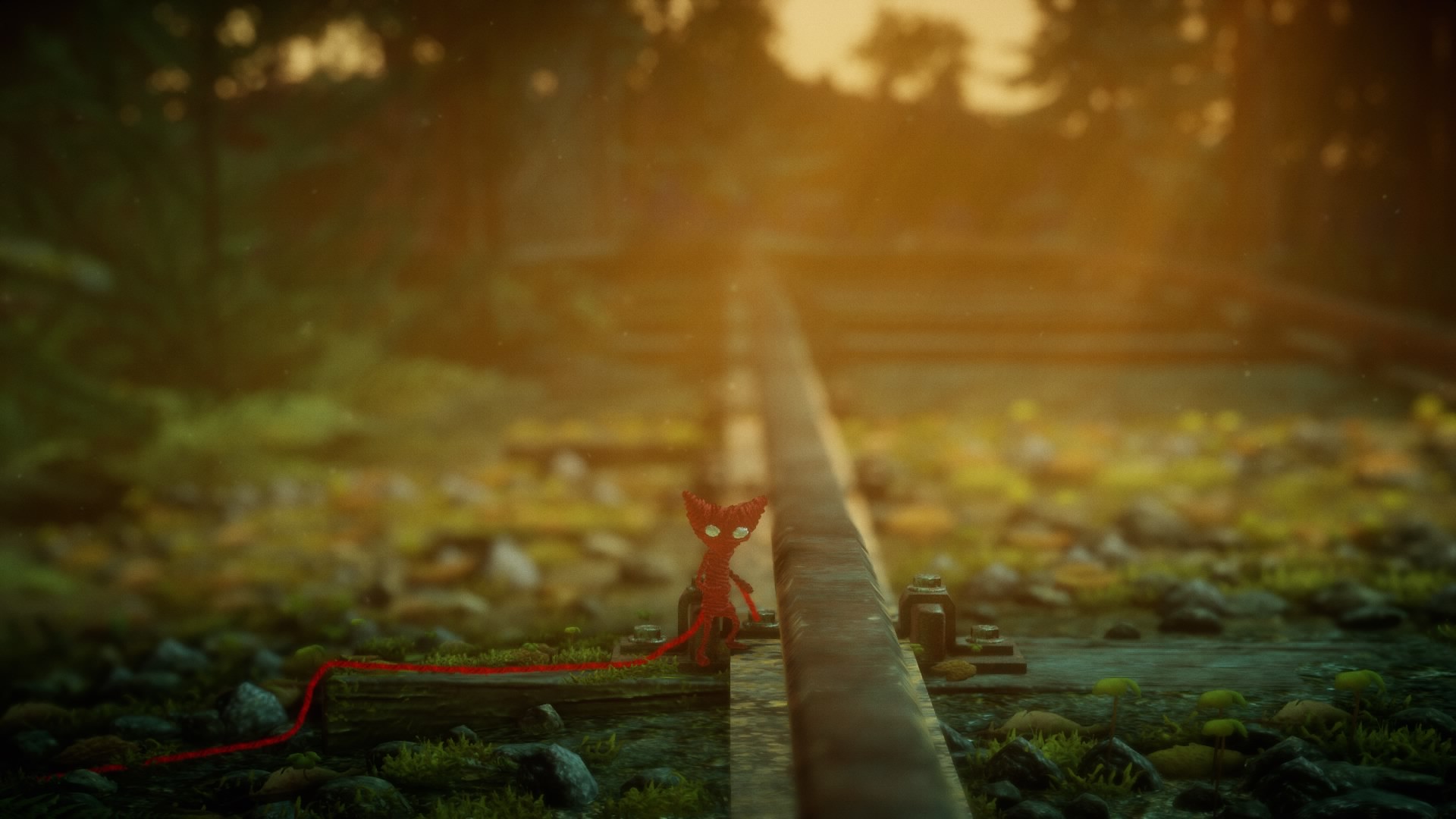In this detailed image from the video game "Unravel," we see a small red character known as Yarny, created from yarn with white-green eyes and ear-like or horn-like features on its head. The character has long limbs and a red cord of yarn extending from its body. Yarny appears to be traversing a railroad track set in an outdoor environment, surrounded by natural elements such as rocks, grass, and trees. The scene is bathed in the warm hues of a sunset, casting a reddish glow over the landscape, which enhances the mystical and fantasy-like ambiance of the setting. The game, published by EA, is known for its co-op gameplay where players navigate Yarny through various challenges in a beautifully crafted world.